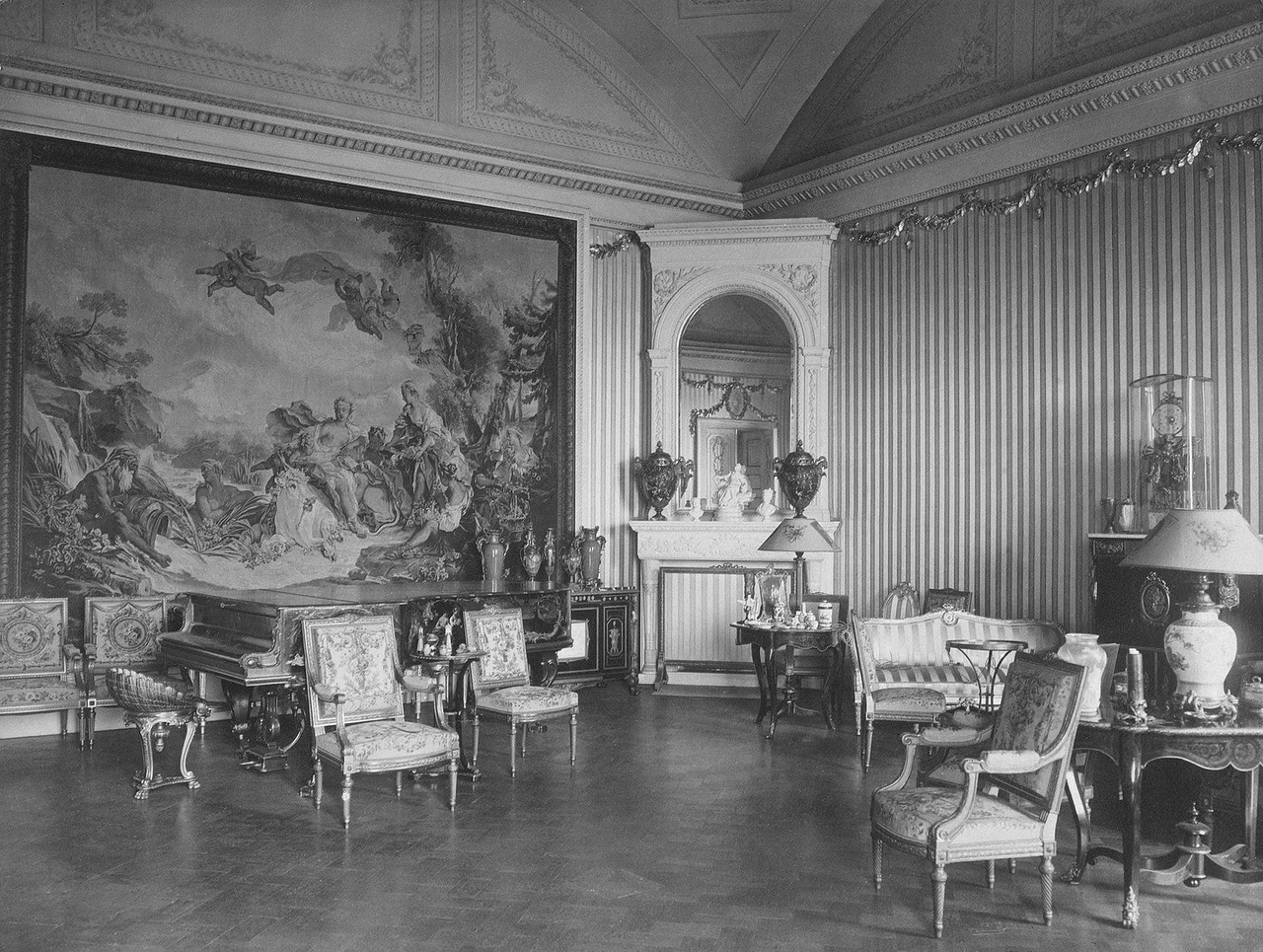This black-and-white photograph, approximately 5 to 6 inches wide and 4 inches high, captures an opulent Victorian-era room, with a focus on the corner of the room. The left wall is adorned with an expansive mural depicting a celestial scene with angels and people at a riverside, extending from floor to ceiling. Beneath this mural resides a baby grand piano with ornate filigree designs and a decorative stool. In contrast, the right-hand wall features vertical gray and white striped wallpaper and is furnished with several stiff, wooden chairs and coffee tables that speak to the period’s distinctive style. Centrally placed in the corner is an elegant piece of furniture with a mirror, shelves, vases, and small statues. The floor appears light gray, possibly wooden or tile squares. The room’s grandiosity is further emphasized by its vaulted and arched ceiling, crowned with lavish molding and metal ribbon-like decorations. This setting evokes the sophisticated yet ostentatious taste of a bygone era, making it reminiscent of a palace or a luxurious estate.